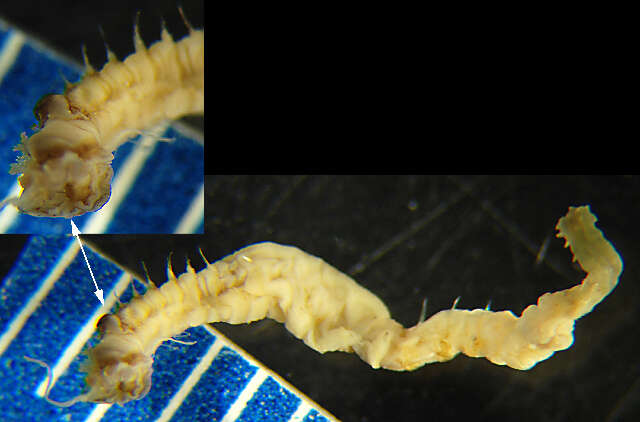This photograph features a pale yellowish-brown, worm-like creature against a predominantly black background. The image is divided into two parts: a larger main section and a smaller inset in the upper left-hand corner. The main section of the photograph shows the entire length of the organism, which has neither visible eyes nor limbs and tapers from a slightly thicker middle to a thinner tail end. Along its back are fine hair-like spines, concentrated near its head, which diminishes in number along the body's length. The creature is positioned against a bright blue mat or ruler, delineated with white, either diagonal or vertical lines, presumably for measurement purposes. The inset provides a zoomed-in view of the creature's head, highlighting its featureless, slightly pointed structure, and includes an arrow pointing downwards to indicate its relation to the larger image below. The background of the photograph, apart from the blue mat, is mostly dark, with the exception of another darker black square in the far left corner.